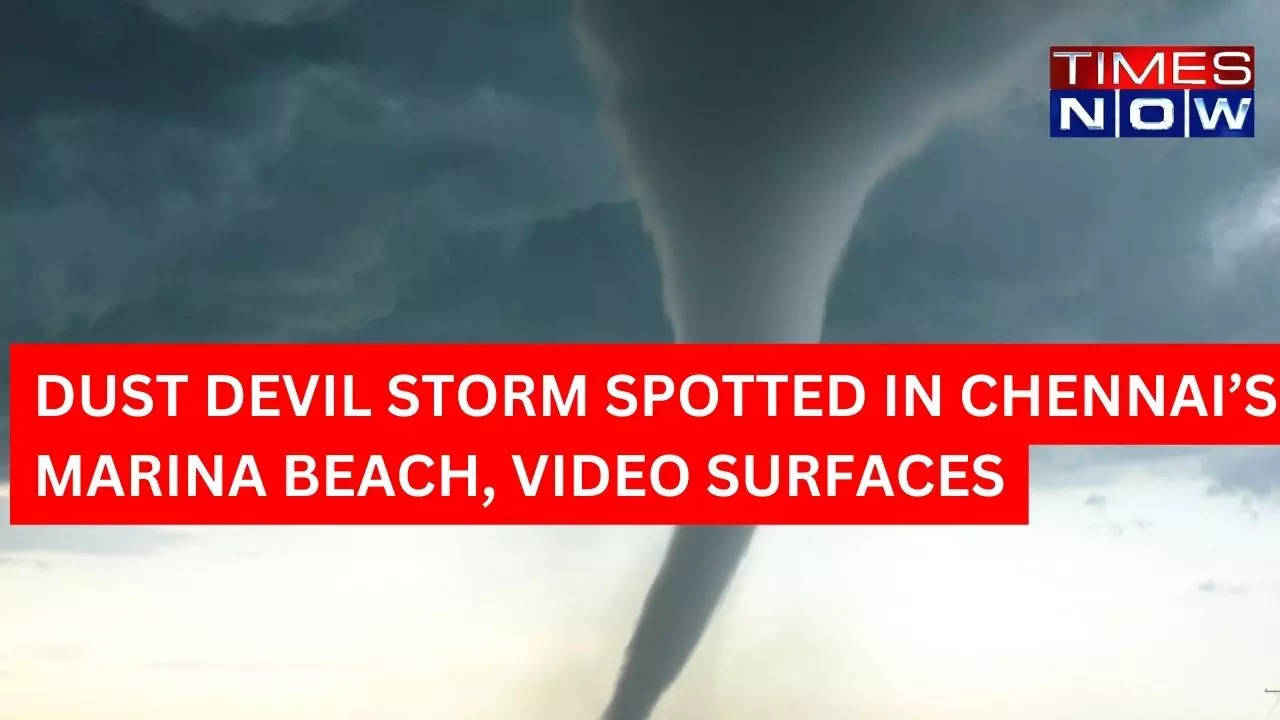This striking rectangular image captures the dramatic scene of a dust devil storm at Chennai’s Marina Beach. Dominating the image is a formidable tornado, its base visible at the bottom of the frame while its swirling gray and blue funnel extends upwards, growing wider and darker until it disappears into a menacing sea of dark clouds. The sky above is densely clouded, enhancing the foreboding atmosphere. A red ticker running across the middle of the image prominently displays the text in white letters: "Dust Devil Storm spotted in Chennai's Marina Beach, video surfaces." In the top right corner, the "Times Now" logo is featured, with 'Times' on a red background and 'Now' on a blue background. The overall impression is one of intense meteorological activity, with the image capturing the raw power and scale of the storm.